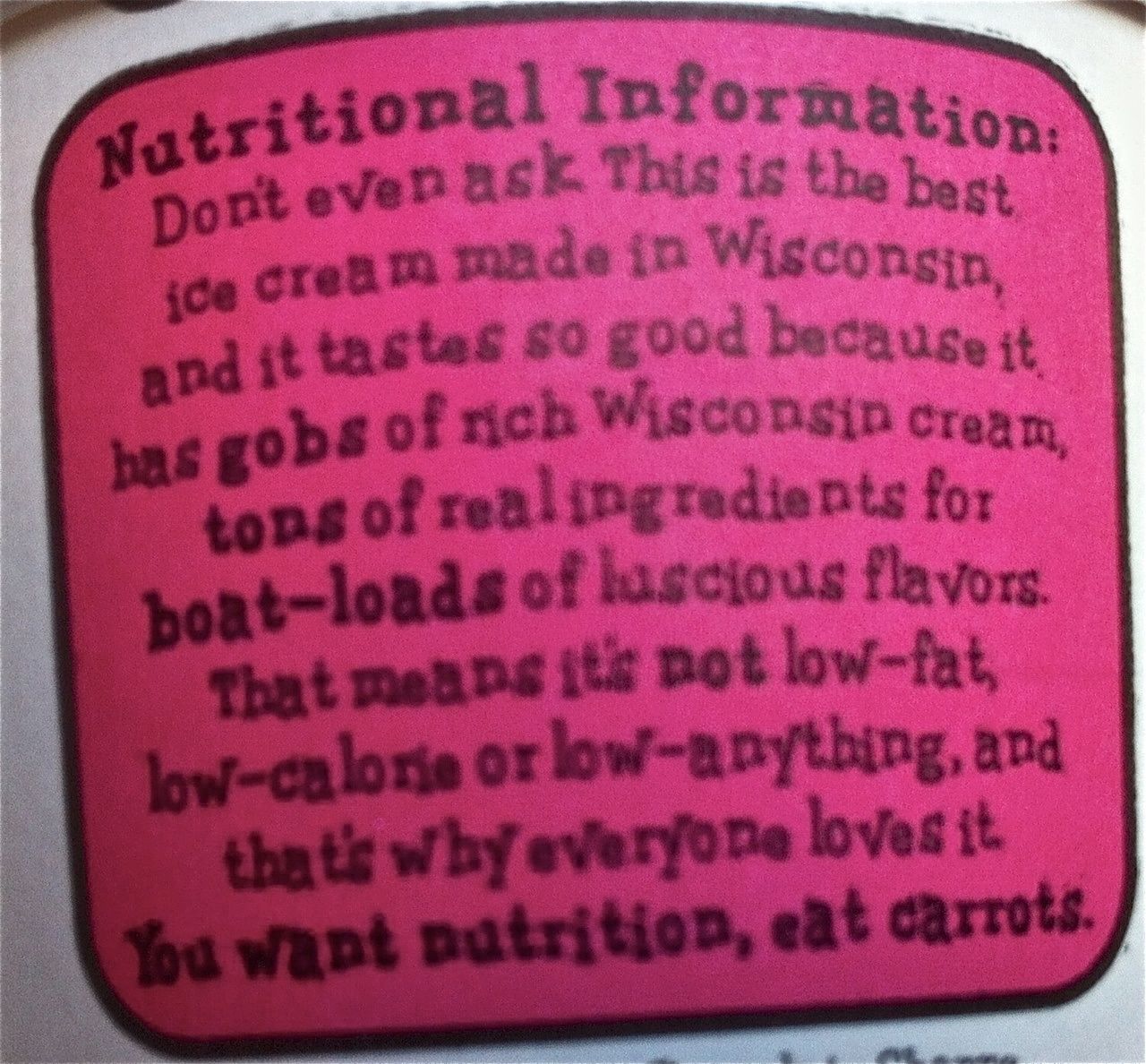This photograph showcases a humorous nutritional information label from a package of ice cream. The label is a bright fuchsia pink square on a white carton, bordered with black. It features playful, bubble-like black text that reads: "Nutritional Information: Don't even ask. This is the best ice cream made in Wisconsin, and it tastes so good because it has gobs of rich Wisconsin cream, tons of real ingredients, for boatloads of luscious flavors. That means it's not low-fat, low-calorie, or low-anything, and that's why everyone loves it. You want nutrition, eat carrots." The witty message emphasizes the indulgent nature of the ice cream, highlighting its rich and flavorful composition.